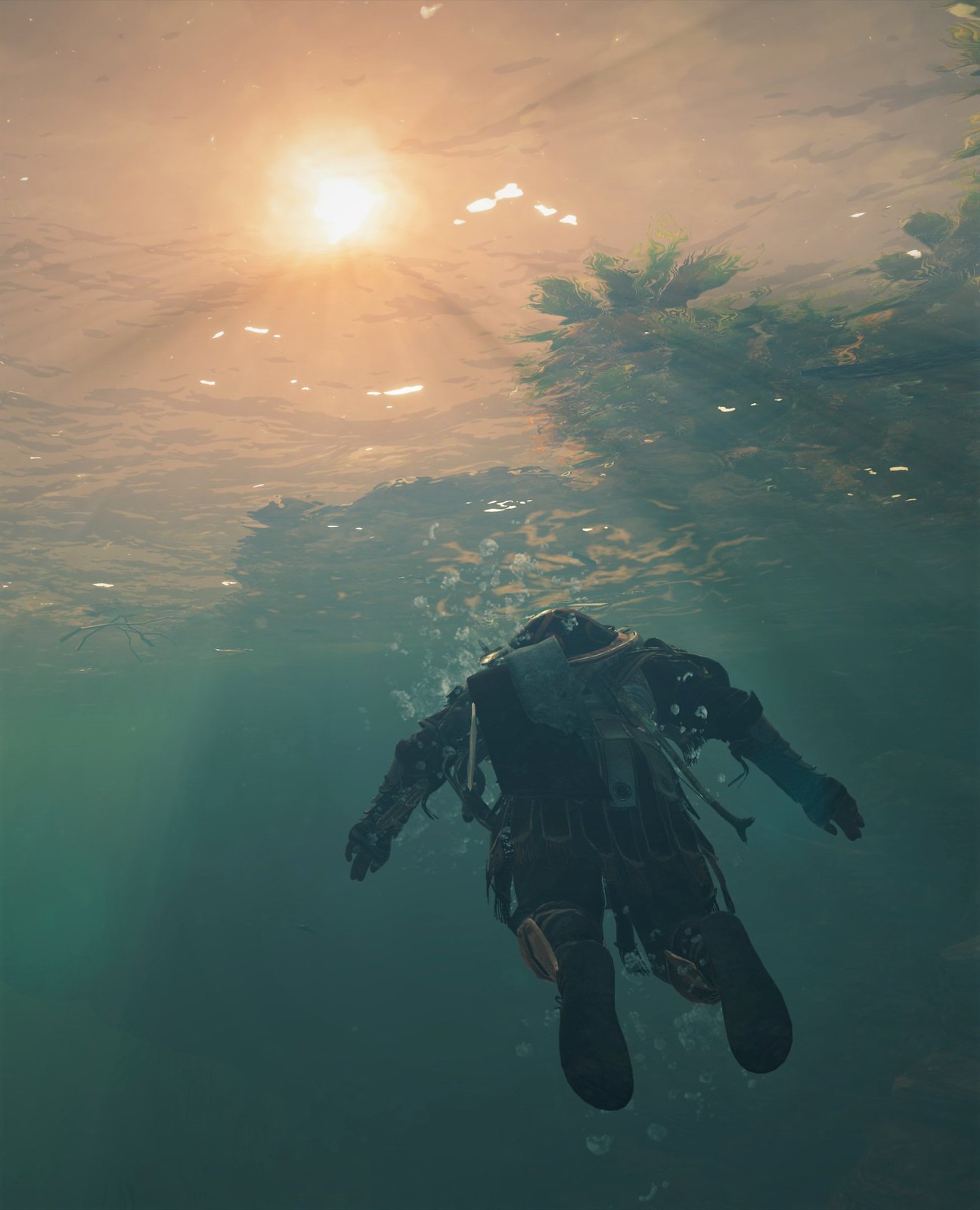In this rectangular image, we see a scuba diver in black gear slowly ascending towards the water's surface, framed by an underwater view looking up. The diver is surrounded by bubbles and is clad in extensive diving equipment, which includes elements that resemble flaps on a tunic and shin guards, adding a gladiatorial feel to the gear. The water is an intriguing mix of colors, with deep green shades below the diver, gradually transitioning into brighter hues as the eye moves upward. At the top left, the sun beams down with bright yellow-white rays, causing god rays to penetrate the water. The area around the sun features a striking orange-peach transition, enhanced by the water's refraction. On the right, the reflection of tree branches, possibly palm trees, distorts through the surface, contributing additional green hues. White speckles, likely from the sunlight filtering through the water, add to the dynamic visual impression.